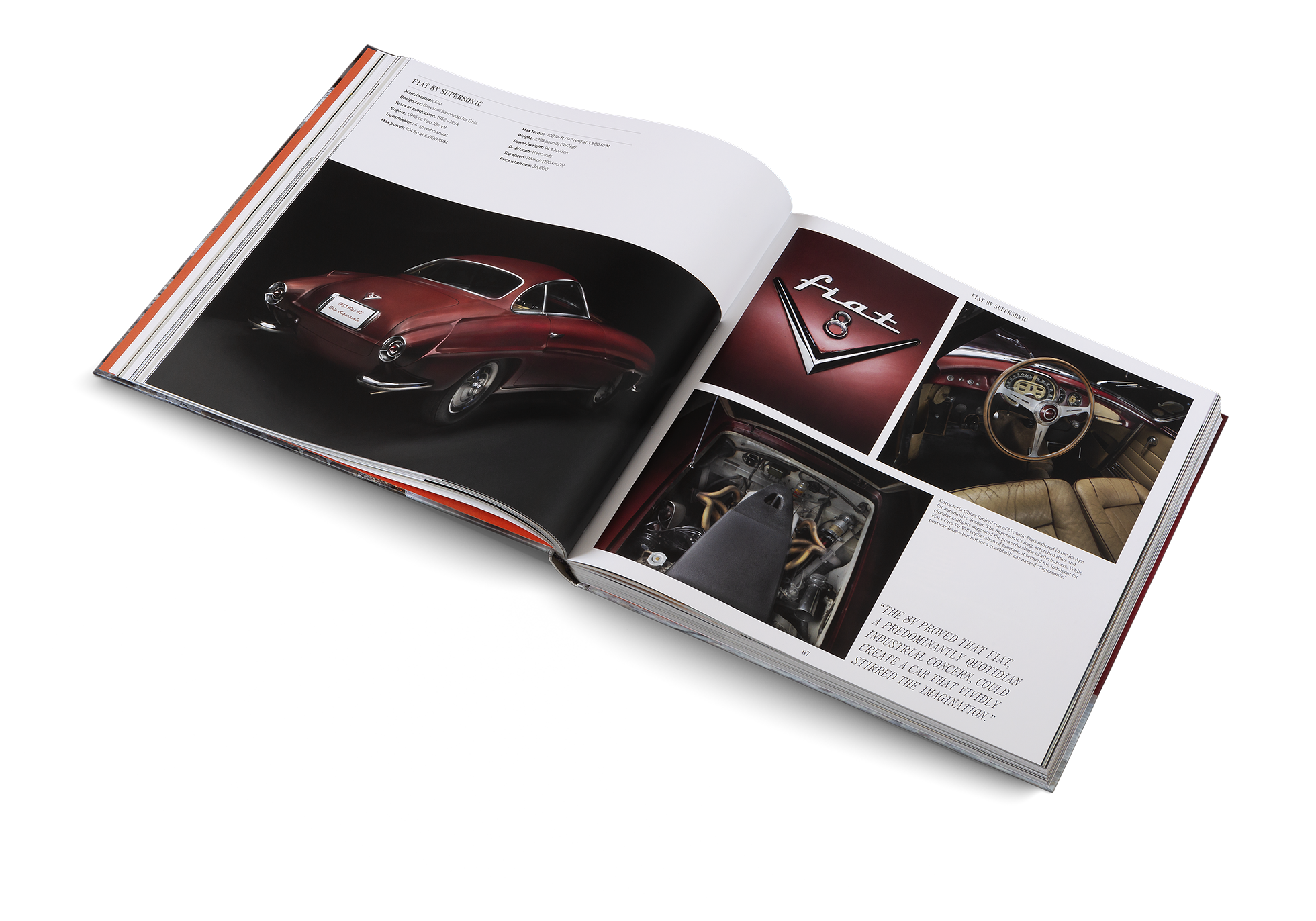This detailed photograph captures an open book showcasing a vintage Fiat car, likely from an era around the 1960s. The book, opened to roughly 20% of its content, is slightly tilted against a stark white background. The left page prominently features a red Fiat 8V Supersonic, viewed from a three-quarter angle. This red, two-door car is bordered by a white frame, set against a dark gradient background. Although most of the descriptive text above is too small to read, key terms such as "Fiat 8V Supersonic" and hints of “max price,” “engine,” “max power,” and "weight" are discernible.

On the opposite page, three distinct images highlight different aspects of the Fiat car. The first image shows the Fiat logo in close-up. The second image provides a detailed view of the car's interior, showcasing tan seats, tan doors, a red dashboard, and a tan and silver steering wheel against a gray or black floor. The third image, located at the bottom right, displays the car's engine, with silver and tan components, accompanied by partially legible text that includes the words "gears" and "Supersonic." The page concludes with a larger, readable caption at the bottom right, celebrating the Fiat 8V: "The 8V proved that Fiat, a predominantly quotidian industrial concern, could create a car that vividly stirred the imagination."